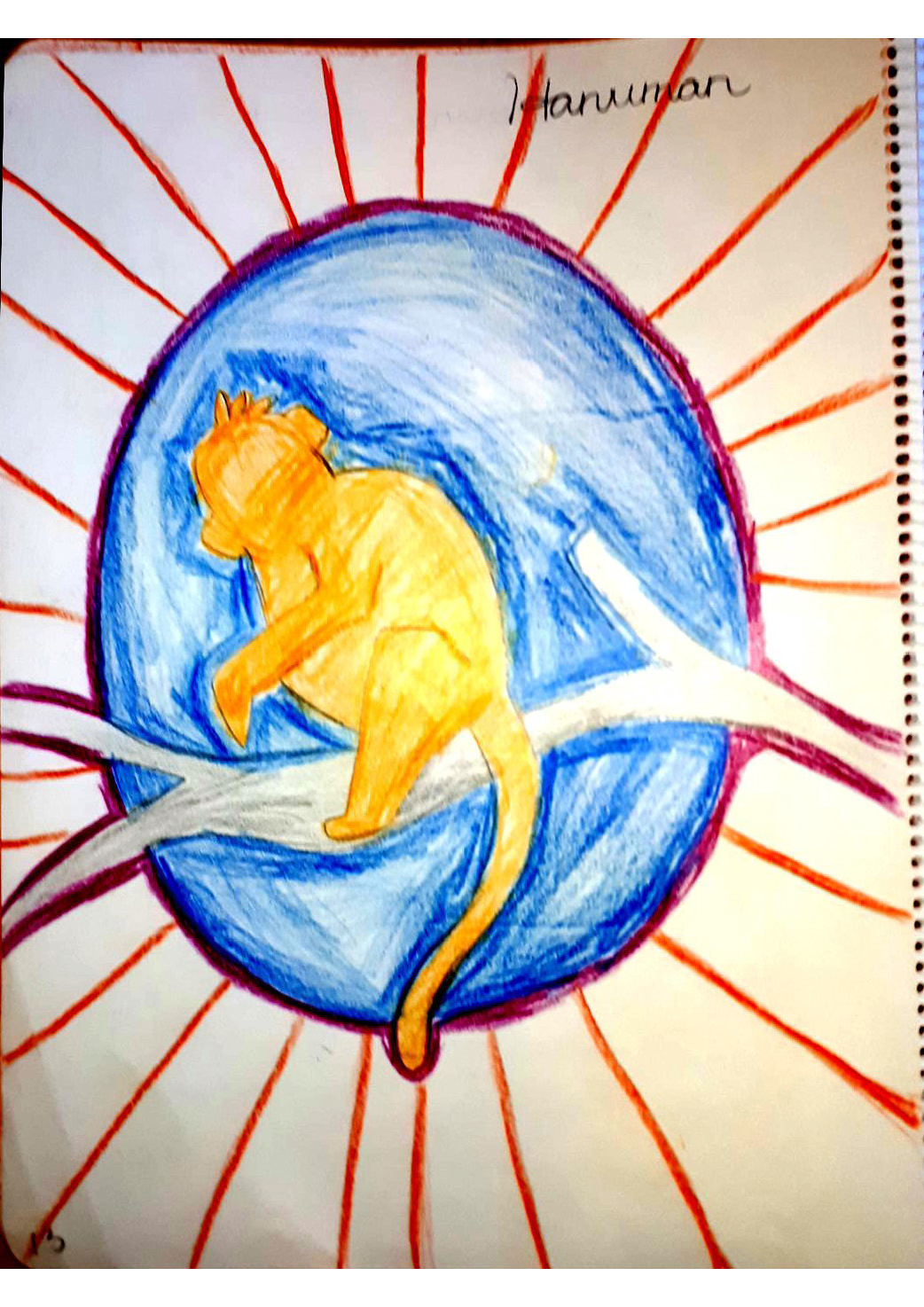The drawing is featured on a notebook page, identifiable by the small holes on the right-hand side through which clear spiral rings are threaded. Central to the image is a large, blue oval outlined in burgundy. Inside this oval, there's an orange monkey depicted with a fine outline, perched on a white and gray branch. Radiating from the oval are red lines, extending symmetrically in all directions. Additionally, the number "13" is visibly marked in black on one of these red lines in the bottom left-hand corner. At the top of the drawing, the name "Hanuman" is elegantly inscribed in cursive script.